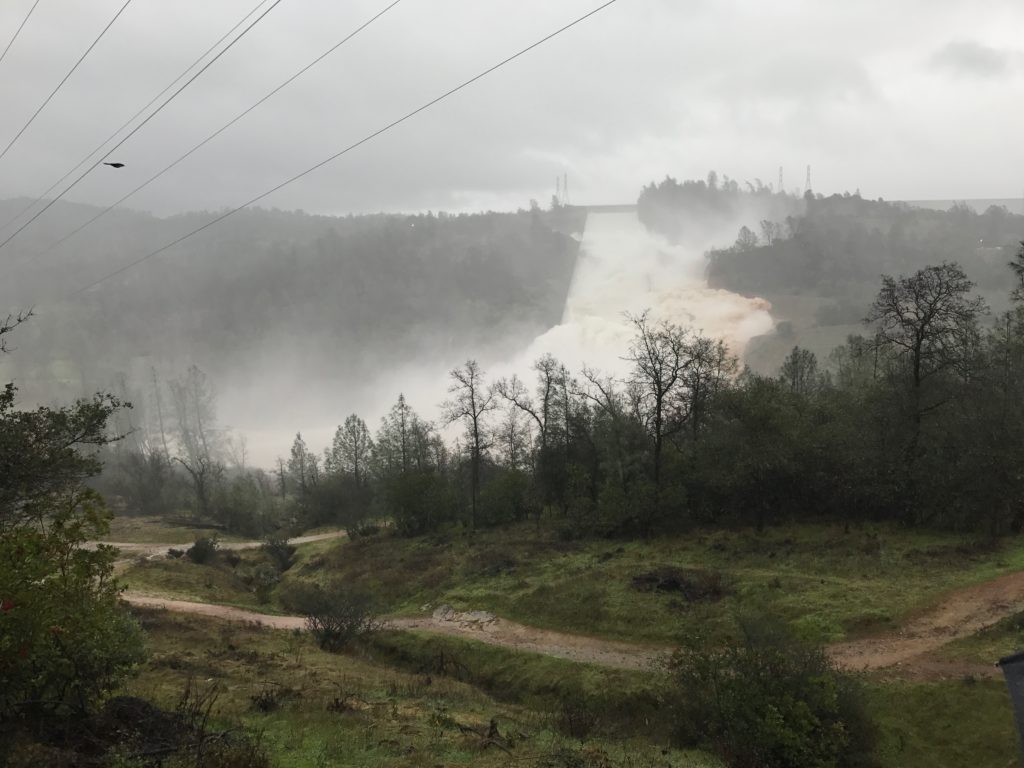A color photograph captures a sweeping landscape on a gray, overcast day. The foreground features a green expanse with various beige dirt paths winding through the grassy area, curving off toward the right. Scattered trees dot the landscape, lending a sense of nature's calm. In the top left corner of the image, power lines are visible but remain unanchored by any discernible power poles. The background reveals a series of hills or mountains, with the most noticeable feature being what appears to be a waterfall or possibly a large plume of smoke, suggesting either a natural water feature or an ongoing accident. This vertical rush of water or smoke cascades down between the hills, creating a focal point that's difficult to clearly define. Interestingly, in the top left, an ambiguous object that some might mistake for a helicopter hovers, adding an additional layer of mystery to this compelling outdoor scene. The photograph is devoid of any people, animals, buildings, or cars, allowing the viewer's attention to focus solely on the natural and potentially catastrophic elements within the frame.